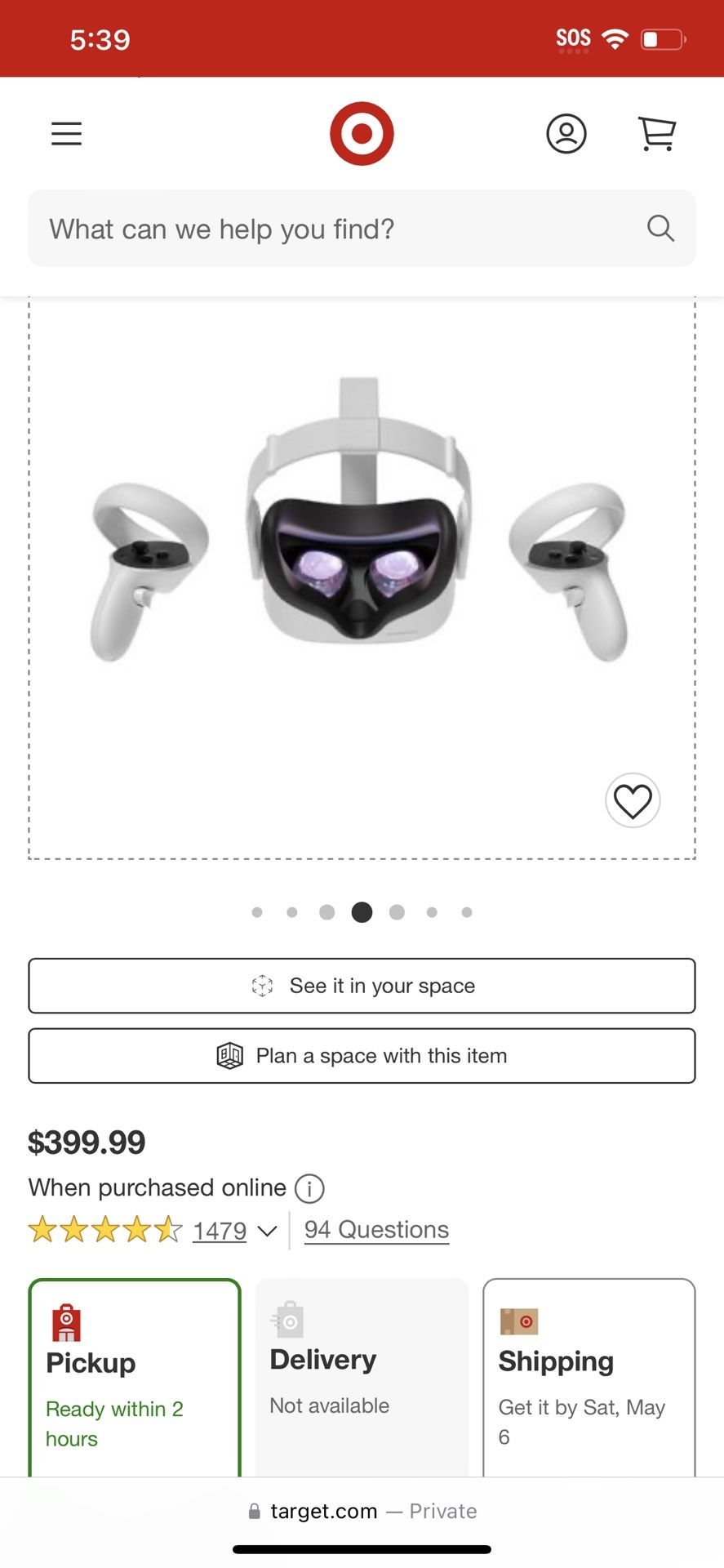A detailed mobile screenshot of the Target website featuring a product page for a virtual reality headset can be seen. At the top, there's a red banner with white text displaying the time "5:39." On the right, indicators show an SOS alert, Wi-Fi signal, and a white square symbol. Below is the main Target web app interface. The top navigation bar includes three horizontal lines (menu icon) on the left, the Target logo in the center, a user icon, and a shopping cart icon on the right.

Directly beneath, there’s a light gray search box with the placeholder text "What can we help you find?" accompanied by a magnifying glass (search icon). Highlighted prominently in the main content area is a photo of the VR headset enclosed in a dotted line, with a like symbol (heart icon) in the bottom right corner. To the right of this image are seven dots, indicating the presence of multiple photos available for selection.

Below the main image are two action buttons: a white box with a black outline labeled "See it in your space" and another similarly styled box labeled "Plan a space with this item." The price is listed at $399.99 when purchased online. Additionally, the product is rated four out of five stars in yellow, based on user reviews, and has 94 questions listed. 

A green-highlighted message indicates the product is "Pick up ready within 2 hours," but delivery is not available. Shipping details state that the item can be shipped by Saturday, May 6th. At the very bottom of the screenshot, the website "target.com" is noted, indicating that the page is being viewed in a private browsing window.